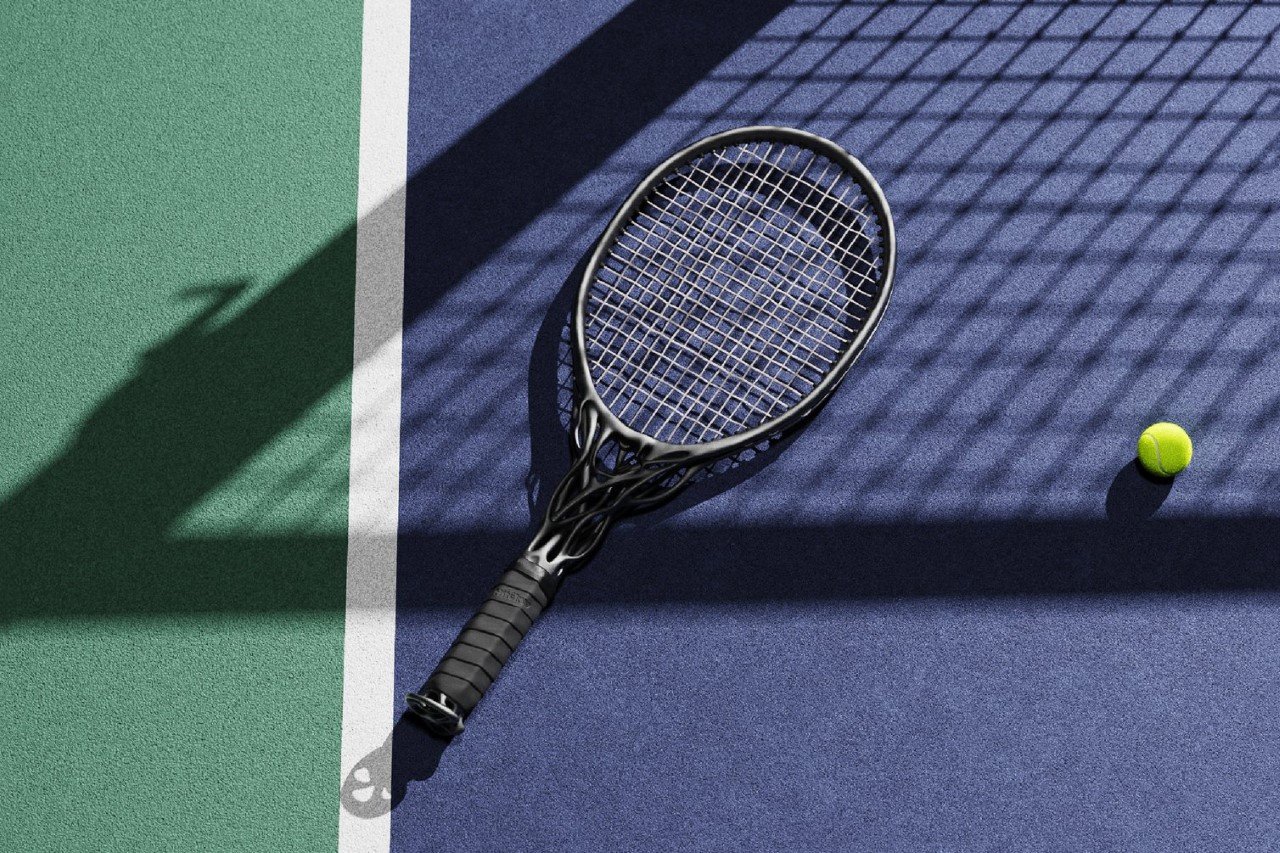The image depicts a tennis court divided into two sections: a navy blue playing surface and a green section, separated by a prominent white stripe. The blue surface occupies about three-quarters of the right side, while the green surface is on the left. The shadows of the tennis net are clearly visible on the court. Positioned diagonally on the blue side is a black tennis racket with a unique design resembling spider webs or muscle fibers on its head and silver strings. The handle of the racket is black. To the right of the racket, closer to the middle of the image, lies a standard bright lime-yellow tennis ball. The image captures the equipment as if they were casually laid down during a match, with the distinct colors and lines of the court providing a vivid backdrop.